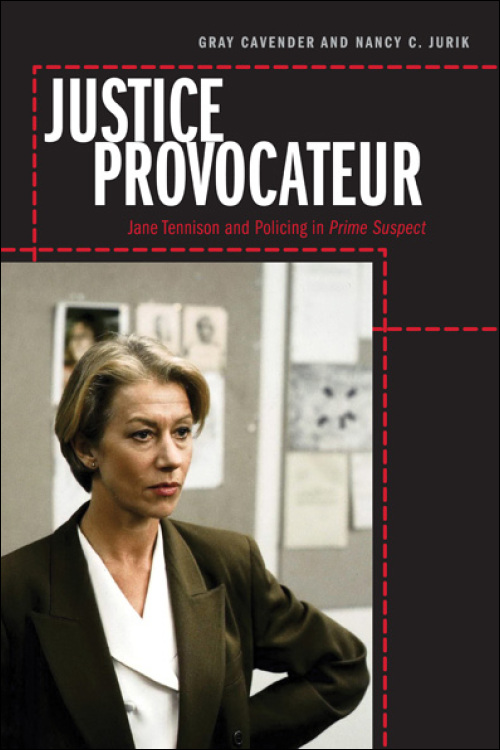This image features the cover of the book titled "Justice Provocateur." The background is predominantly black, providing a stark contrast to the text and imagery. At the top, the authors' names, Gray Cavender and Nancy C. Jurik, are prominently displayed. Below that, in bold red font, is the subtitle "Jane Tennyson and Policing in Prime Suspect."

Dominating the left two-thirds of the image is a figure of a woman, depicted in a confident stance. She is dressed in a white shirt paired with an olive green suit coat, and her left arm rests assertively on her hip. The woman has a short haircut, conveying a sense of professionalism and determination. Behind her, there is a backdrop featuring images of cop dramas, adding context and depth to the subject matter of the book. The design effectively combines textual and visual elements to evoke a sense of intrigue and authority related to law enforcement themes.